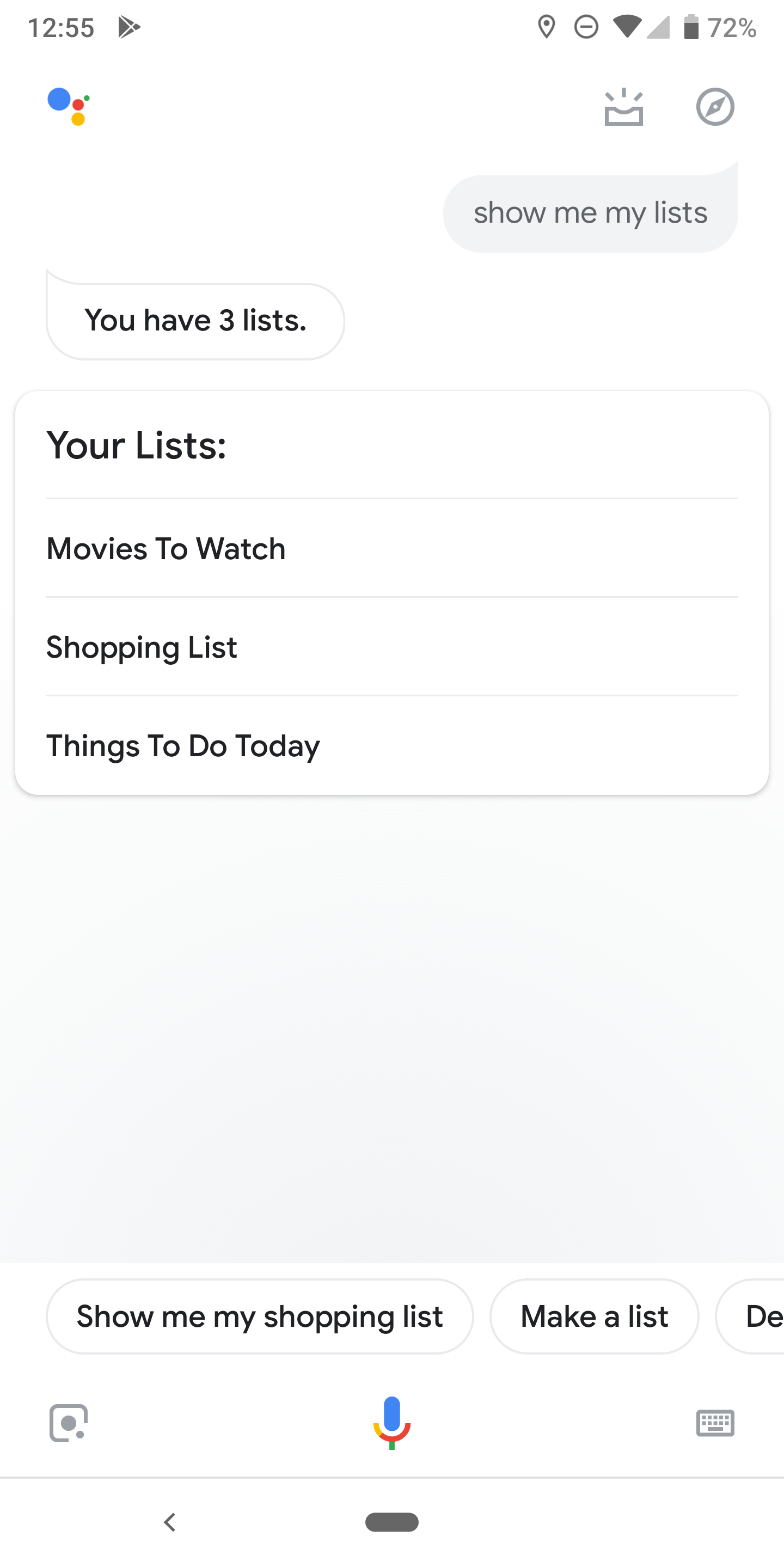The image captures a smartphone screen exhibiting the "Your Lists" section of an application. 

At the top left corner, the time is displayed as 12:55. To the right of the time, there is a series of status icons, including a Wi-Fi icon, a connection icon, and a battery percentage icon indicating the battery is at 72%. 

Below this status bar, on the left side, there are two gray icons accompanied by a small blue, red, and yellow dot. 

Further down, to the right, there is the text "Show me my lists" displayed prominently. Underneath this, in black text, there are three list names in a separate section titled "Your lists": "Movies to Watch," "Shopping List," and "Things to Do Today." 

Below this section, there is a light gray square background containing suggestions, such as "Show me my shopping list" and "Make a list."

At the bottom of the screen, three icons are visible:
- A camera lens icon on the left.
- A microphone icon in the middle.
- A keyboard icon on the right.

Finally, a small gray bar is centered at the very bottom of the screen. The rest of the background around these elements is white, providing a clean and minimalistic appearance.